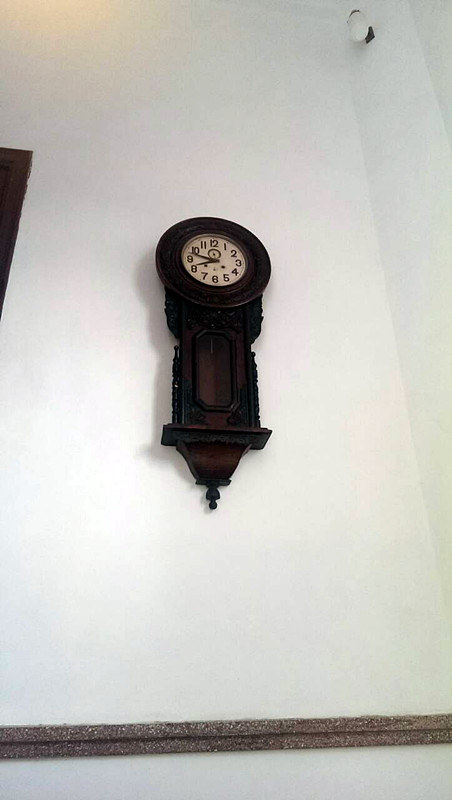This photograph features a distinguished clock mounted on a white wall, complemented by a gray chair rail that runs horizontally along the wall's midsection. The clock, crafted from dark wood, exhibits a classic design with a circular top and a pointed bottom adorned with a finial. Its tan face is marked by slender hands, indicating the time is approximately 9:40. The elegant simplicity of the white wall and gray chair rail provide a sophisticated backdrop, highlighting the clock as both a functional timepiece and an ornamental element in the room.